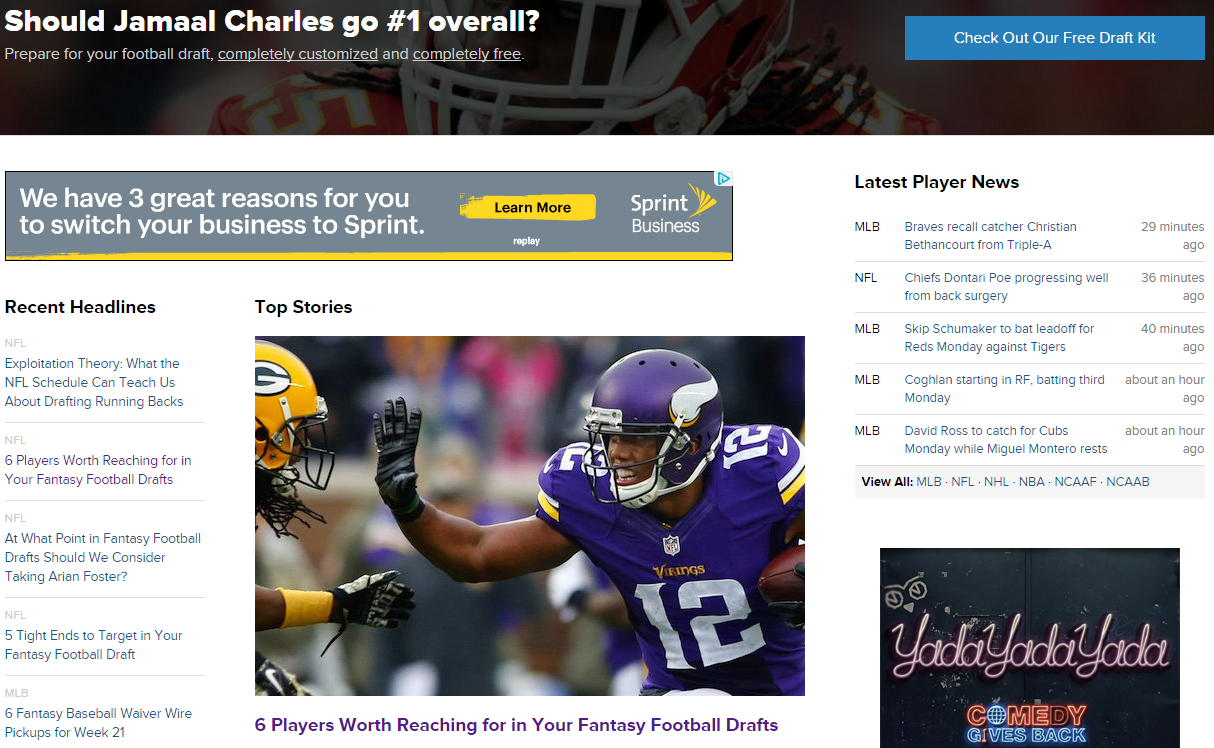This detailed caption brings clarity and organization to the original description of the fantasy football website screenshot image:

---

The image displays a screenshot from a fantasy football website in portrait orientation, slightly wider than it is tall. At the top, white text poses the question, "Should Jamal Charles go number one overall?" Below this, smaller white text reads, "Prepare for your football drafts completely customized and completely free," with the phrases "completely customized" and "completely free" underlined for emphasis. To the right, a blue rectangular button with white text prompts users to "Check out our free draft kit." The background subtly features a semi-transparent image of Jamal Charles in motion, with his helmet on and glancing sideways.

Beneath this section, a white-bordered area displays a Sprint advertisement at the top. To the left, headlines are listed with the second one reading, "Six players worth reaching for in your fantasy football draft." The center features the prominently labeled "Top Stories," accompanied by an image depicting a Minnesota Vikings player wearing jersey number 12 attempting to stiff-arm a Green Bay Packers player. Below this image is another headline, "Six players worth reaching for in your fantasy drafts." 

To the right, a column titled "Latest Player News" provides updates on various players from MLB, NFL, and MLB leagues. Further options for sports leagues are available at the bottom, including clickable links for NHL, NBA, college football, and college basketball.